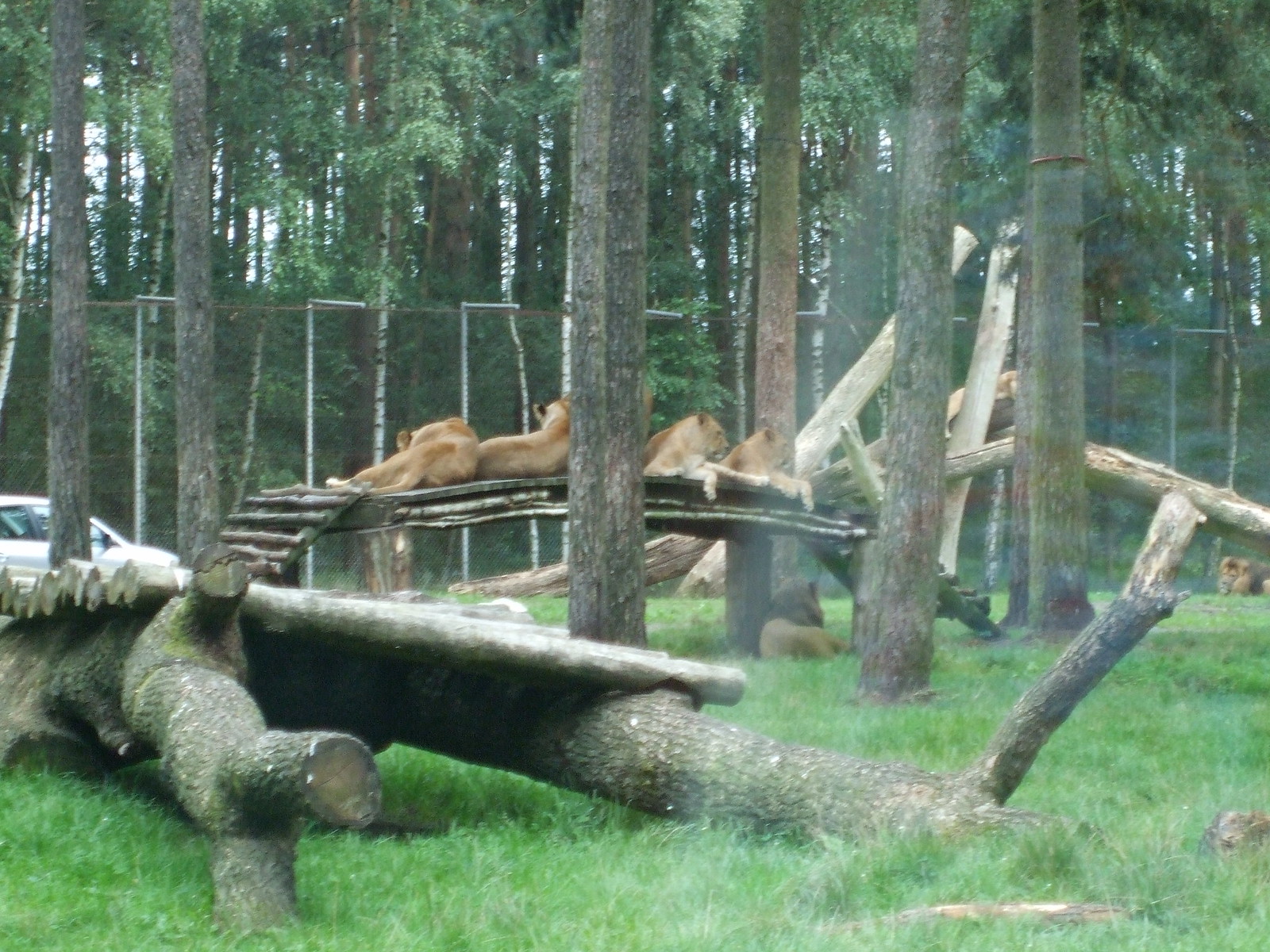The image depicts a lion enclosure, likely in a zoo or wildlife preserve, with a high fence surrounding the area. Amongst the wooded setting with several thin birch trees, six lions are visible lounging in various places. Four female lions rest on a wooden bridge made of downed tree trunks and large branches, which stretches from the foreground into the distance. The first two lionesses are lying with their backs toward the viewer, looking into the distance, while the other two face forward, gazing to the left. A tree separates the pairs of lions on the bridge. Below the bridge, a single male lion with a discernible mane is lying down. In the upper right background, another lioness sprawls on a log, while on the far right, another male lion sleeps beneath a different log. The enclosure is grassy, interspersed with numerous trees and logs providing a naturalistic habitat. Additionally, to the left, outside the fence, there's a car parked, indicating human access to this area.